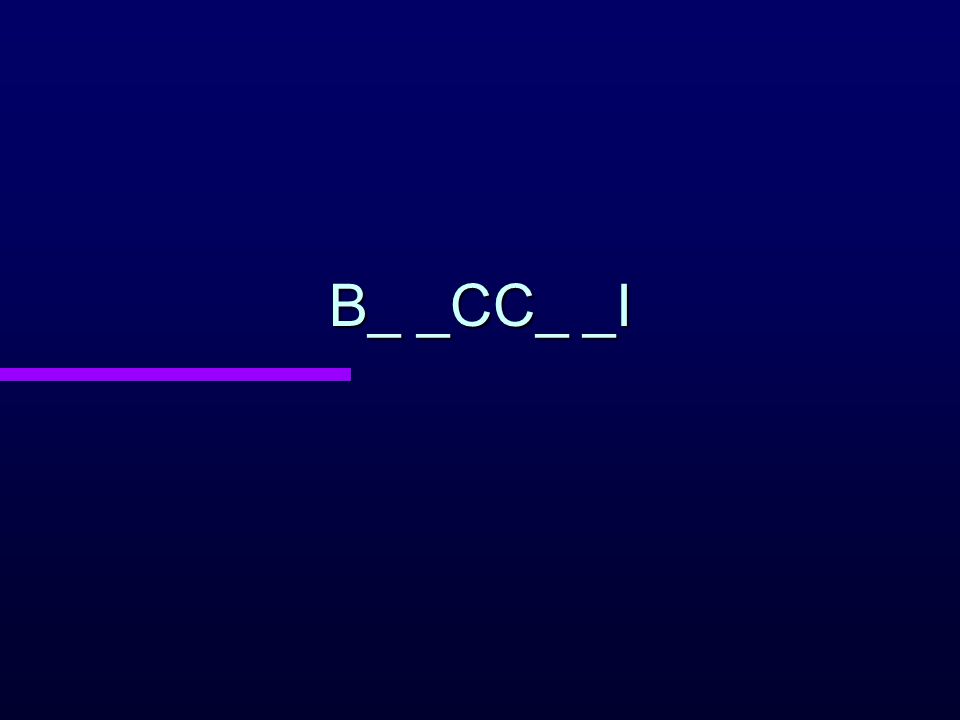The image depicts a dark, gradient blue screen transitioning from a lighter blue at the top to an almost black hue at the bottom. At the center of the screen, both vertically and horizontally, there is a sequence of white uppercase letters and underscores that read "B__CC__L." Situated below this text is a horizontal, narrow purple rectangle, extending from the left edge toward the central region and aligning under the initial letter 'B.' The screen is devoid of any additional images, text, or website references, emphasizing a minimalist layout with the letters and line as the focal elements.